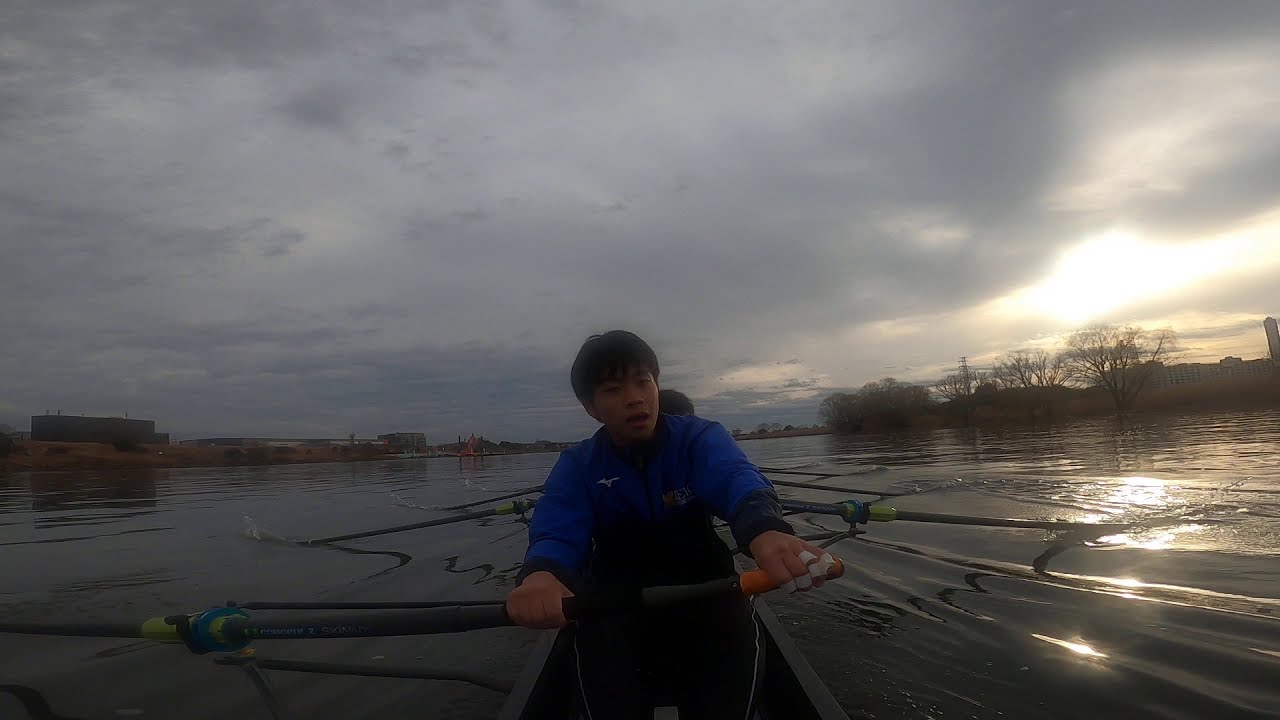In the image, a young individual, possibly in their teenage years and of Asian descent, is paddling a thin black rowboat on a calm river or small lake. The serene water reflects the diminishing light as the sun sets, casting a greyish hue across the scene, partially obscured by dark, heavy clouds. The person, dressed warmly in a blue jacket and black pants, holds a grey paddle with black supports in their left hand, which is wrapped in white tape over several fingers. Although the focus is on the young rower at the front, additional oars can be seen behind him, suggesting the presence of at least one more person whose head is barely discernible. Along the right bank, bare trees line the water's edge, hinting at the cold and overcast weather, while faint outlines of buildings can be spotted in the far left background. The overall ambiance evokes a tranquil yet somber evening, with the stillness of the water and the impending dusk emphasizing the isolated beauty of the scene.